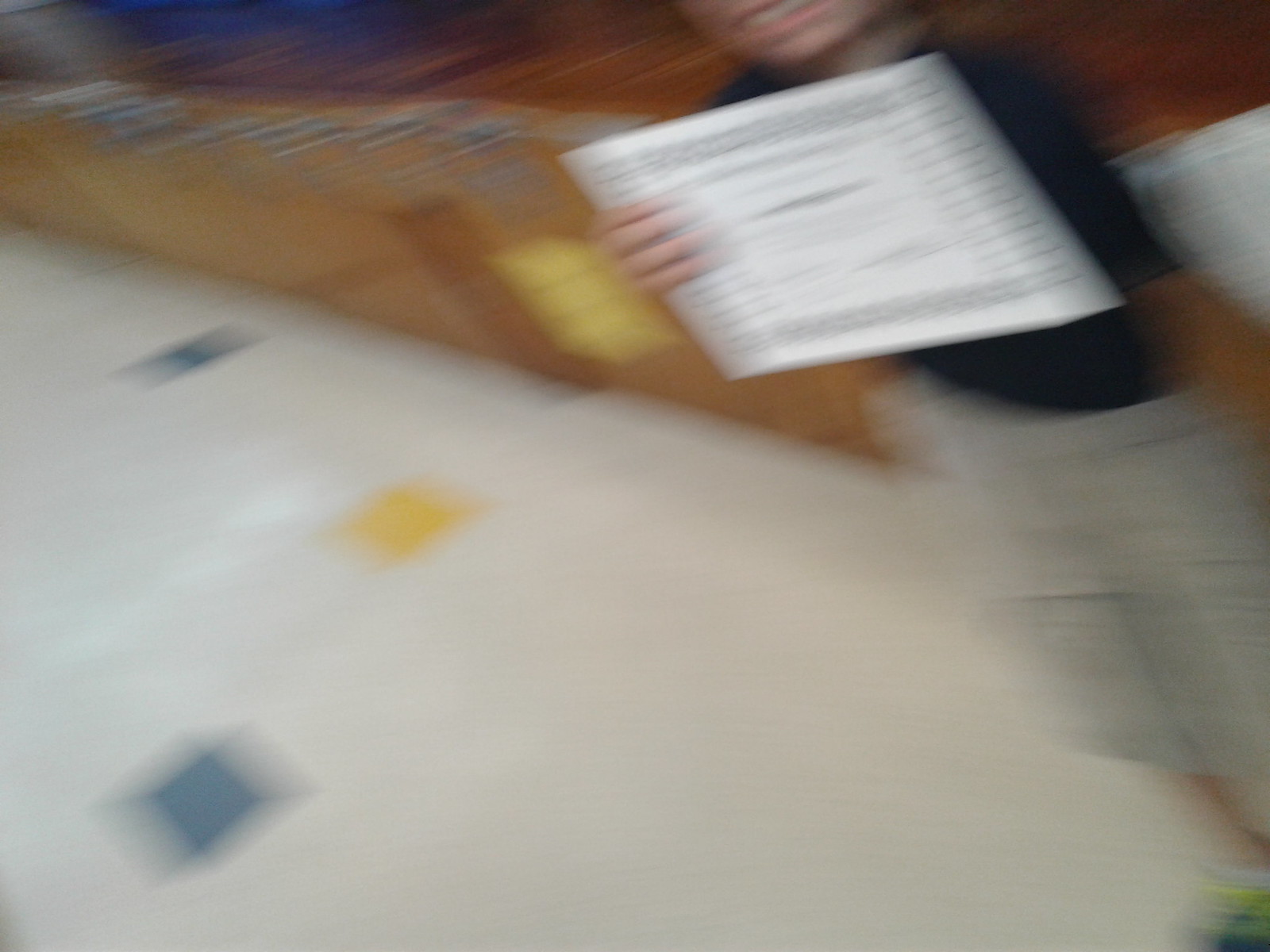The image is a blurred photograph capturing a person who appears to be holding a sizable white certificate with a bronze design along its edges in their right hand, close to their face, as they read it. The person is smiling, indicating happiness about the certificate they received. Even though the image is very blurry due to possible movement, the person's smile, including their teeth and lips, is visible, though specific facial features like eyes and nose are not clear. The individual seems to be dressed in a dark black shirt, grayish-tan khakis, and bluish-green shoes. They stand on a mostly white tile floor interspersed with blue and yellow tiles. In the background, there is a wooden stage, some brown tables, and other indistinct details, underscoring the hurried or dynamic nature of the photograph.